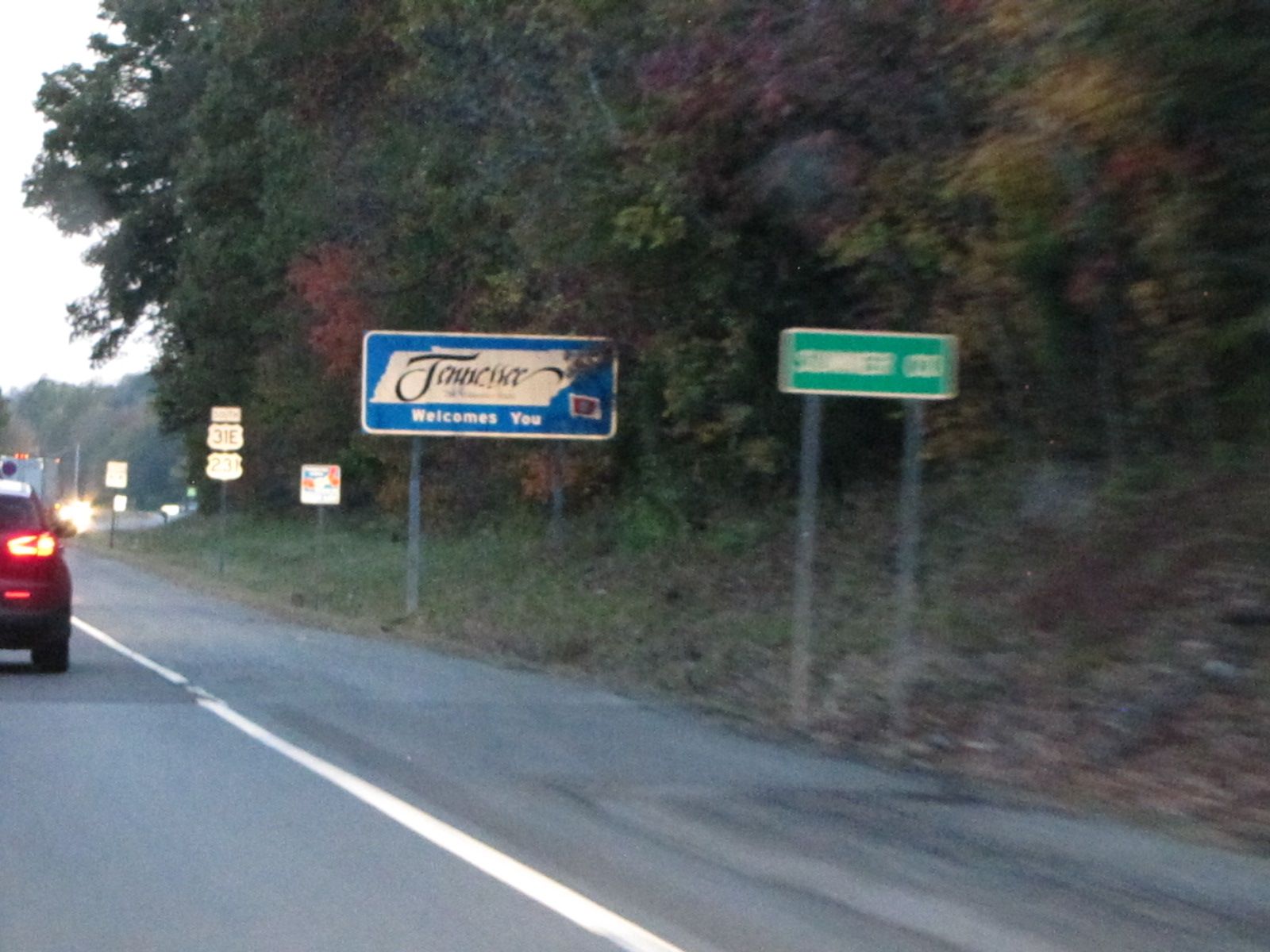A color photograph captures a scenic outdoor view along a highway in Tennessee. The image, slightly blurry and out of focus, depicts a gray asphalt road marked by a white stripe on its right side. Adjacent to the road, a grassy, dirt-covered slope rises, leading to a backdrop of trees adorned with green, brown, and light brown leaves. Prominently in the foreground, a red car drives by. Further down the road, signs indicate the location: one rectangular sign features a map of Tennessee with the words "Tennessee welcomes you" written in script, and another green sign with a white border, though too blurred to read. On the opposite side of the road, street lights and additional signs hint at the approach of dusk or early morning, as oncoming vehicles have their headlights on.